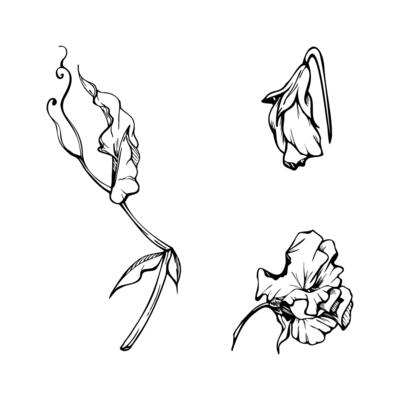This black-and-white line drawing, rendered in either black pen or charcoal pencil, resembles an illustration from a botanical guide for identifying herbs and plants. It features three distinct images of a flower at various stages of its lifecycle, all presented against a white background.

On the left, there is a long-stemmed flower with two downward-pointing leaves, accented by two curly vine-like structures in the background. The flower itself, situated on the top right of the stem, has a profile view and appears more rectangular than round.

In the top right section of the illustration, the flower is shown in a wilted state, hanging from a bent stem reminiscent of a cane top. The bloom is sagging and looks forlorn, emphasizing a stage of decay.

Finally, the bottom right displays the flower in its full, healthy bloom. This view reveals a lush array of petals spreading outward, curling slightly, and converging into a central point, much like a lily. Each of the right-hand illustrations features partially visible stems, contrasting with the fully visible stem in the left-hand depiction.

Overall, the drawing captures the flower's lifecycle in a clear, if somewhat simplified, style that allows viewers to recognize each stage from blossoming to wilting.